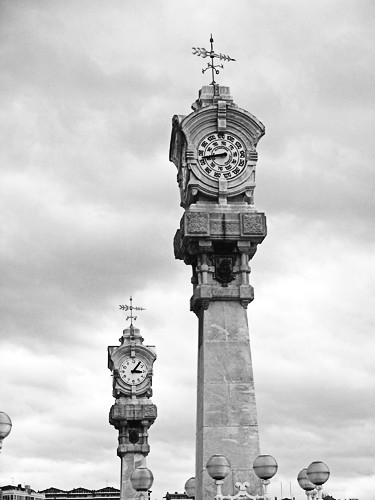This black-and-white photograph captures a picturesque view of two distinct, Celtic-style stone clock towers. Both towers, meticulously crafted from gray mortar and brick, emanate a sense of timelessness with their elaborate ornamental details and tiered stone layers. The prominent tower in the foreground features a heavy stone face adorned with a mechanical barometer, distinguished by its air pressure dial, and crowned with a weather vane indicating the cardinal directions: north, south, east, and west. This clock shows the time as quarter to nine. Not far off, in the background to the left, another similarly designed tower stands tall, its clock displaying the time as five after nine. Both clocks and barometers are showcased within grand archways, enhancing their majestic appearance. The sky overhead is densely clouded, adding a dramatic backdrop to the intricate stonework and enhancing the photograph's timeless and somewhat ethereal quality. The image perfectly marries the elements of timekeeping and weather forecasting, set against an architectural testament to timeless craftsmanship.